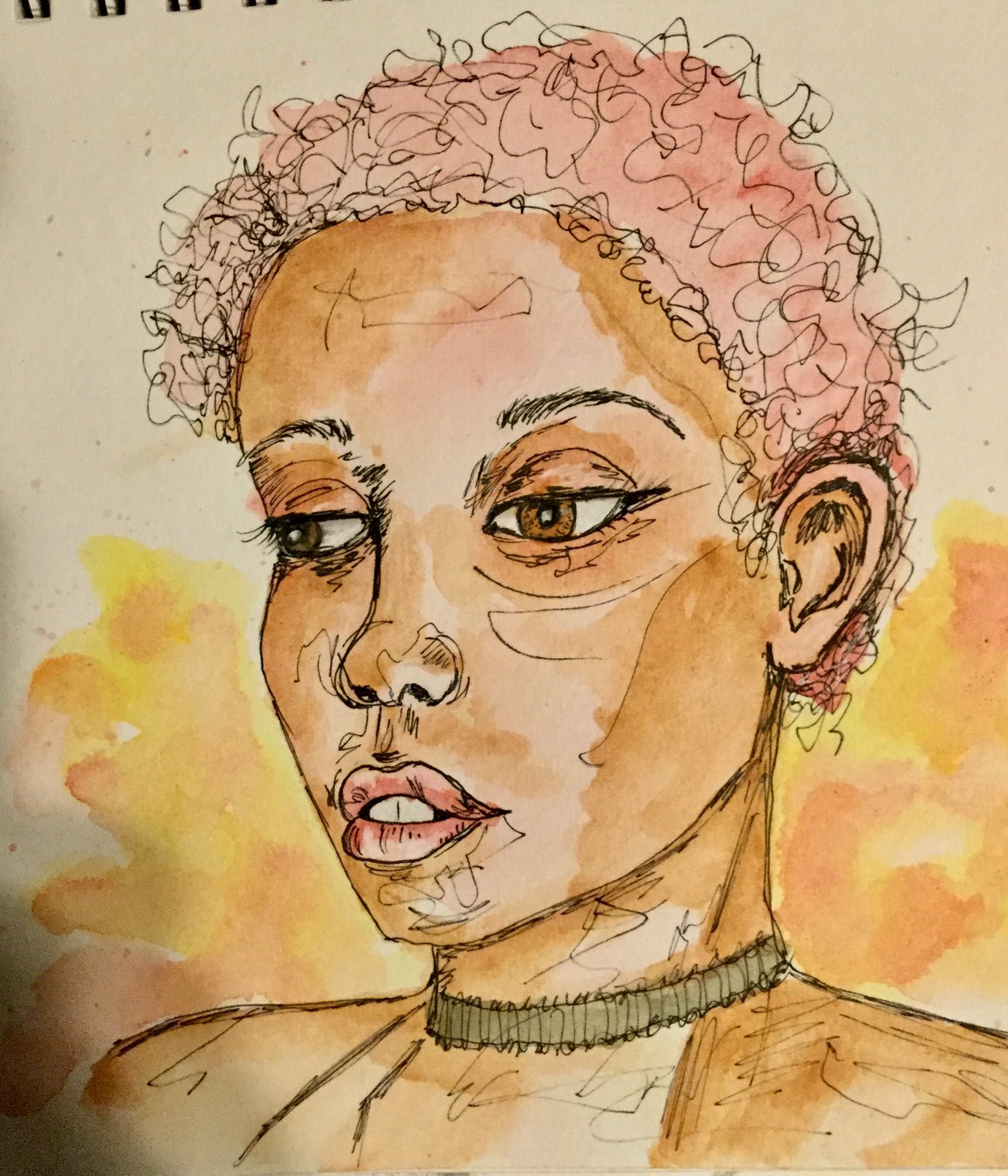This image is a detailed pen and ink and watercolor illustration on a white drawing pad or watercolor paper that's spiral-bound at the top, as evidenced by the visible spiral bindings at the top left. It depicts an African American woman with finely sketched and inked features. Her hair is illustrated in pink watercolor with black squiggly lines throughout, giving the appearance of curly hair. The woman's face is presented in a slight left profile, though the right side is still visible.

Her expressive face is adorned with large, beautiful brown eyes with dark, inked eyebrows and long eyelashes. There are various shades of tan and brown watercolor highlighting her light brown complexion, accompanied by pink hues on her forehead and around her ear, suggesting a light to medium brown skin tone. Her slightly parted lips reveal her teeth, and there are subtle ink markings around her nose and mouth, as well as along her neck and shoulders for additional texture and detail.

The illustration includes a green choker necklace snugly fitting around her neck, contributing to the character's stylish appearance. The background is enhanced with a light wash of watercolor in yellow, pink, and tan, framing her face from just beneath her eyes down to her shoulders, creating a delicate, blended effect that helps her figure stand out against the white page. This watercolor wash appears watery and fluid, adding to the overall softness and depth of the piece.